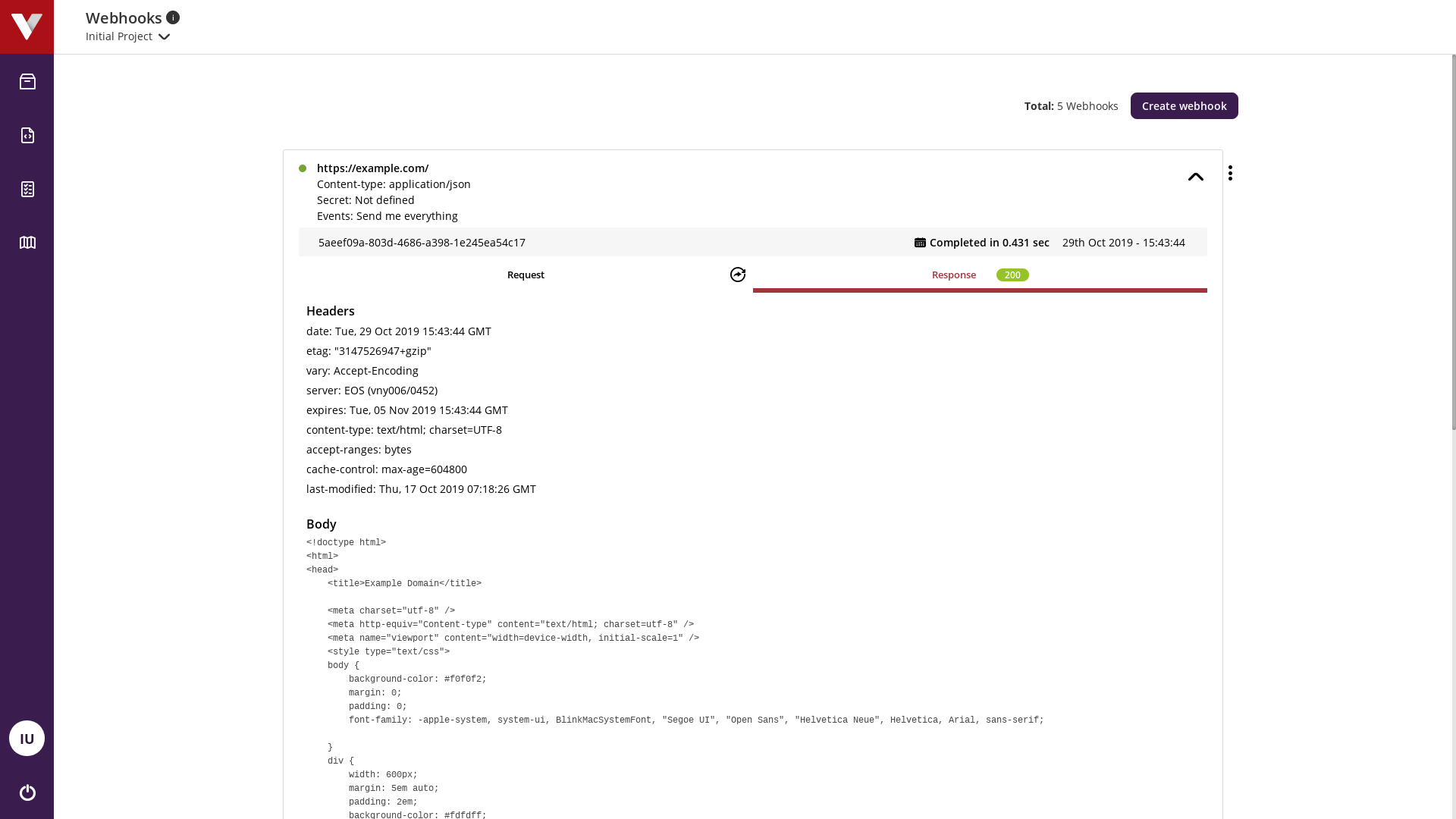This image is a detailed screenshot of a webhook request details page from a project dashboard. The layout is clean, organized, and divided into several main sections for easy navigation.

- **Top-Left Section**: 
  - Project Name: "Initial Project"
  - Title: "Webhooks"
  - Total Count of Webhooks: 5
  - Action Button: "Create Webhook" for adding a new webhook.

- **Main Content Section**: 
  - The section prominently displays the details of a specific webhook request.
  - **Webhook URL**: `https://example.com`
  - **Content Type**: `application/json`
  - **Secret**: Not defined
  - **Event Subscribed To**: "Send me everything"
  - **Request ID**: `5aeefo9a-803d-4686-a398-1e245ea54c17`
  - **Status**: Completed in 0.431 seconds
  - **Timestamp**: 29th October 2019 at 15:43:44
  - **Response Code**: 200 (indicating success)
  - **Headers Included**:
    - Date
    - ETag
    - Server
    - Expires
    - Content Type
    - Accept-Ranges
    - Cache-Control
    - Last-Modified

- **Additional Details**: 
  - The page contains basic HTML structure and some CSS styling.
  - **Sidebar**: Located on the left side, featuring various icons, likely for navigation, though their specific functions are not detailed.

The overall design and layout are clean and well-organized, facilitating an easy understanding of webhook details and navigation through the dashboard.